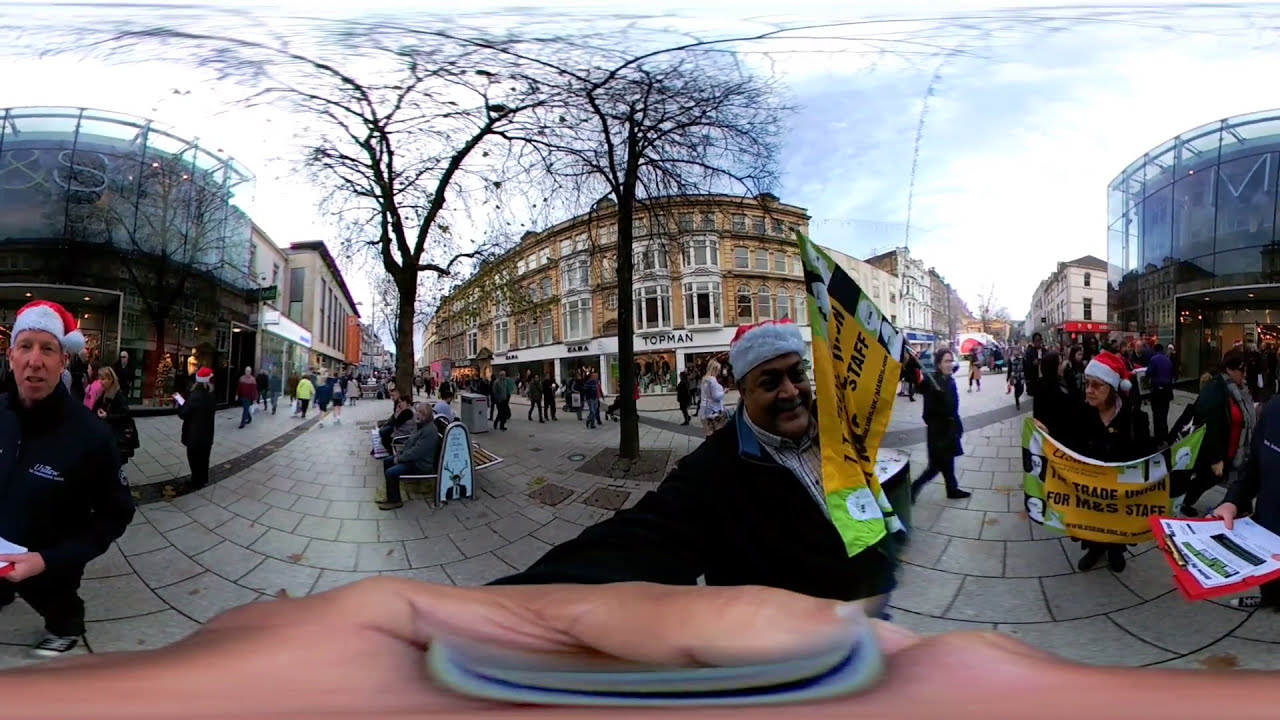The vibrant photo captures a bustling town center, likely located outside an English-speaking country. Taken with a fisheye lens, the image's unique distortion enhances the lively atmosphere of a busy downtown area. The scene is set on a bright day, possibly in the evening, as indicated by the numerous pedestrians dressed in jackets and Santa Claus hats, hinting at a festive season. The ground is paved with smooth, gray stone tiles, and features scattered benches and multiple trees, including a couple of barren ones.

Central to the image is a rotund man wearing a black jacket and a Santa hat, holding a yellow flag adorned with several letters. Flanking him are two other men, also in Santa hats—one on the left appears to be speaking, while the one on the right holds another yellow sign, potentially indicating a protest or petition drive. Amid the crowd, a person with a red clipboard and paperwork stands to the right, possibly gathering signatures.

The backdrop consists of various rounded-edge and apartment-style buildings, including a notable glass building featuring the letter "M". Among the storefronts, a "Topman" retail store is explicitly mentioned. The scene is animated with the hustle and bustle of people, capturing the essence of a lively urban setting.